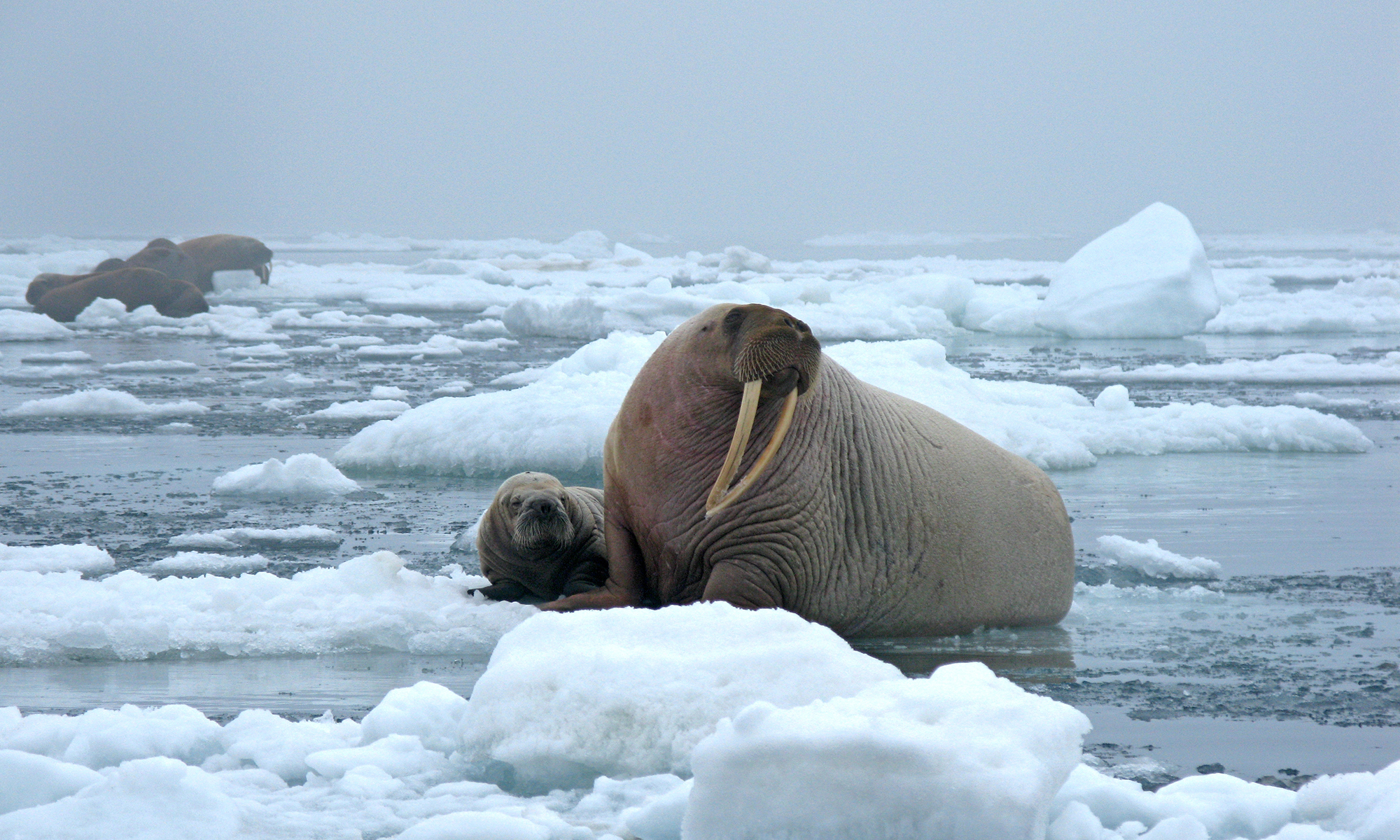This vibrant color photograph, captured by a wildlife photographer, presents a majestic walrus, accompanied by its cub, in a serene and icy landscape. The massive walrus, with its prominent, downward-curving ivory tusks and wrinkled brown body, dominates the foreground as it looks off to the left, seemingly focused on something out of frame. Beside it, a smaller, tuskless baby walrus mirrors its gaze. The entire scene is set amidst a frozen expanse blanketed with thick ice blocks, mounds of snow, and a misty, grey-blue sky. In the background, additional walruses can be seen reclining on the icy surface, partially obscured by the fog and snow. The area exudes a sense of cold, with scattered snow and ice chunks enhancing the wintry atmosphere. A distinctive large ice rock marks the back right corner of the composition, adding yet another layer to this captivating glimpse into the walrus' icy habitat.